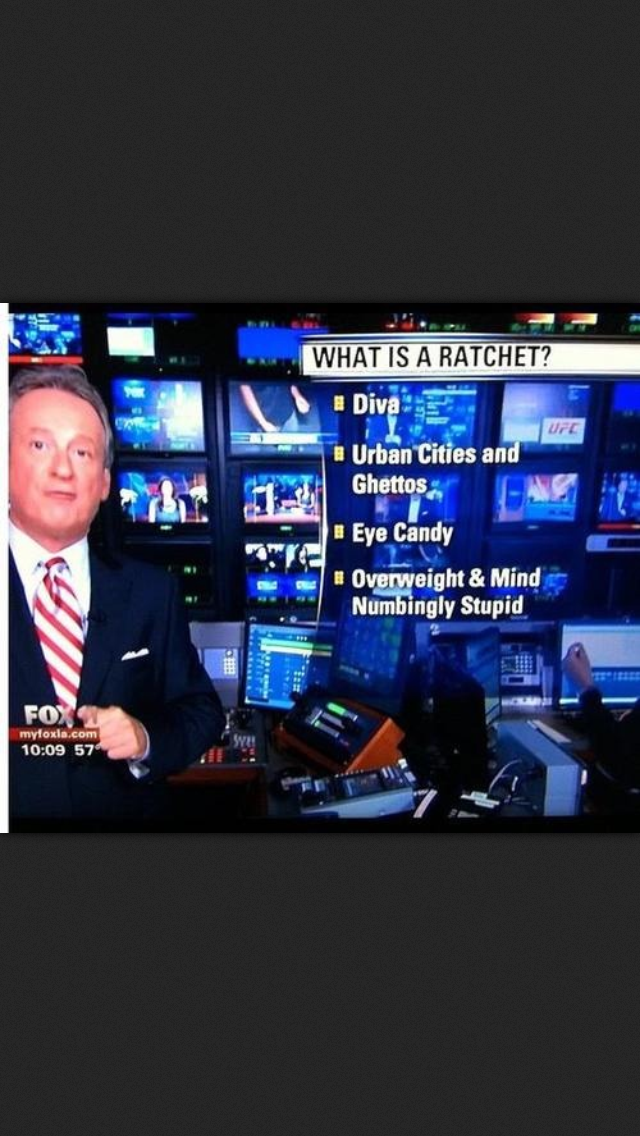The image is a detailed screen grab from a Fox 11 news broadcast. The screen is bordered by black rectangles on the top and bottom. In the bottom left corner, the screen displays the Fox logo, the URL myfox.com, the time 10:09, and the temperature 57 degrees. Dominating the left side of the screen is a man in a business suit with a red and white striped tie, dressed as a news anchor. He has gray hair and appears to be in mid-speech, with his lips pressed close together. To the right of him is a graphic overlaid on the screen. At the top of this graphic, in black text, is the question "What is a ratchet?" Below this, in white text with yellow bullet points, are four descriptors: "diva," "urban cities and ghettos," "eye candy," and "overweight and mind-numbingly stupid." The backdrop of the broadcast resembles a control room wall filled with televisions.